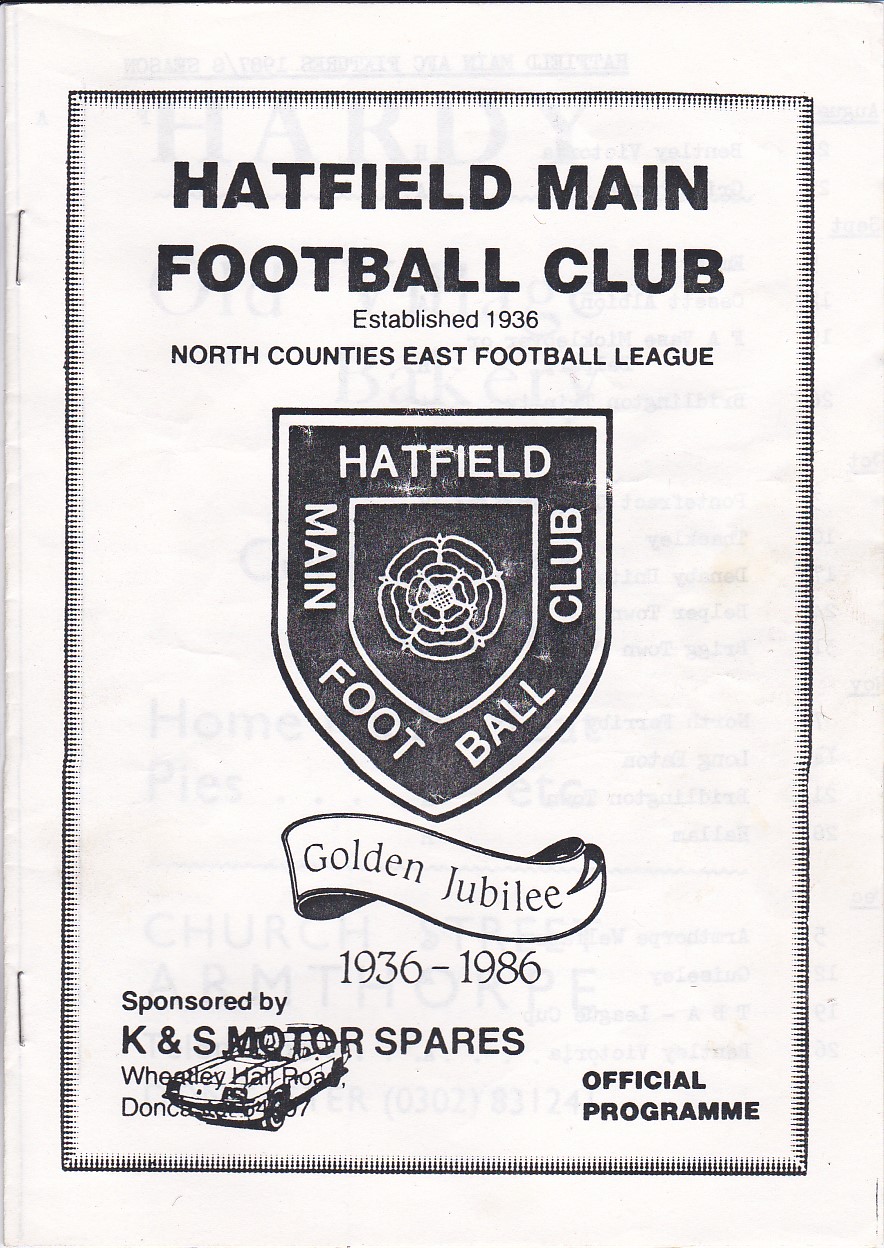The image is of a vintage football program cover for Hatfield Main Football Club, which was established in 1936 and is part of the North Counties East Football League. The cover features a prominent black rectangular border filled with dots that gradually decrease in size. At the top, in bold black letters, it reads "Hatfield Main Football Club" with the establishment year "1936" and league information. Below this, there is an emblem shaped like a shield that also says "Hatfield Main Football Club" and displays a flower symbol in the middle. Beneath the emblem is a white ribbon banner proclaiming "Golden Jubilee 1936-1986." Further down, the text reads "Sponsored by K&S Motor Spares, Wheatley Hall Road," although part of this text is obscured by an illustration of a car. In the bottom right corner, it states "Official Program." The paper has aged well but is thin, allowing the text from the other side to partially show through. There are two staples on the left side holding the pages together.